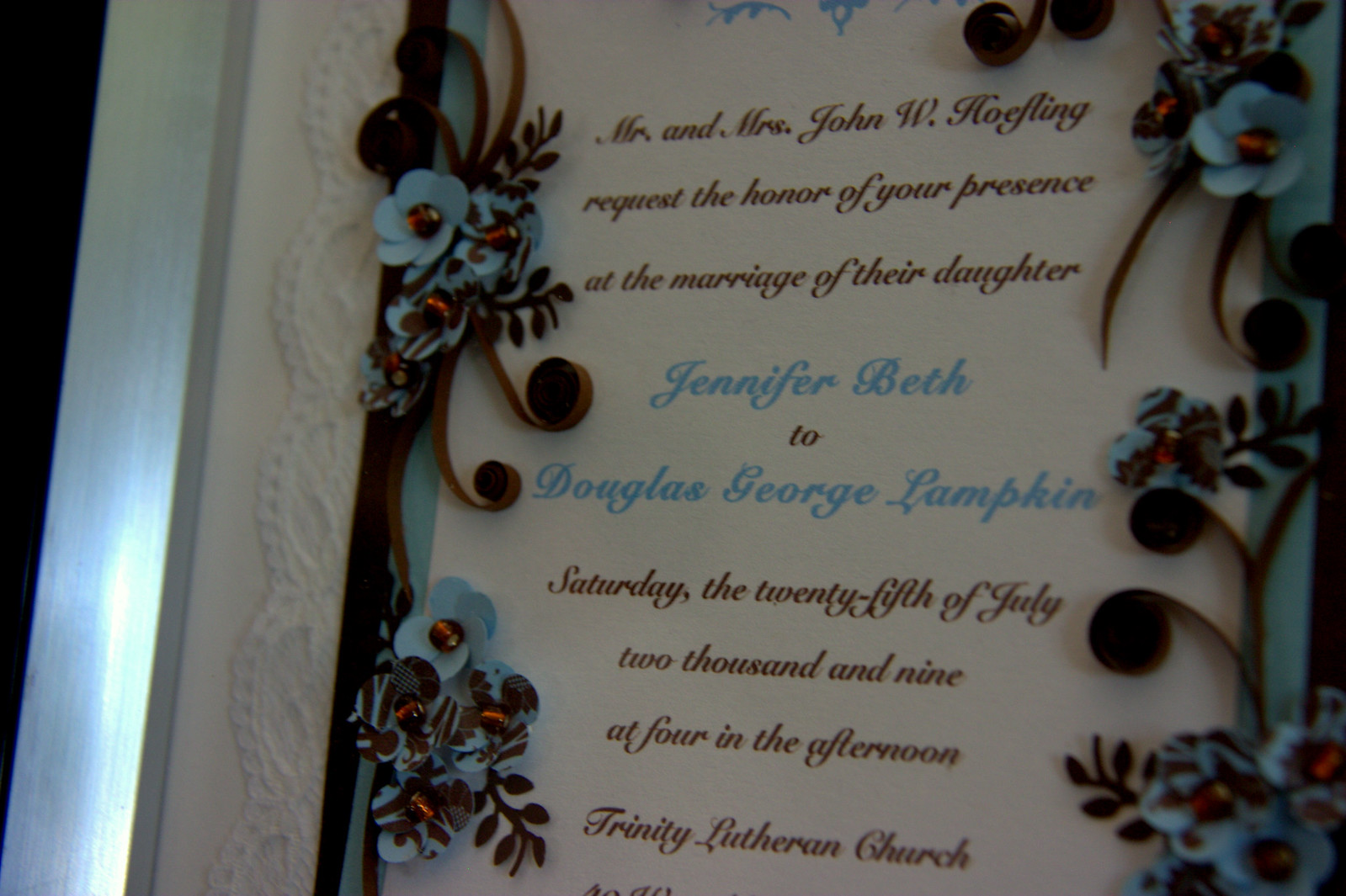In this dimly lit image, there is a cream-colored card, which could also be white due to the lighting. The card features elegant brown cursive lettering that reads, "Mr. and Mrs. John W. Hofling request the honor of your presence at the marriage of their daughter." The names "Jennifer Beth" and "Douglas George Lamkin" are printed in blue script. Below, in brown letters, it states, "Saturday, the 25th of July, 2009, at four in the afternoon, Trinity Lutheran Church," although the text about the location is cut off.

The card is beautifully bordered by delicate baby blue paper flowers with brown trimmings and curled brown leaves, all intricately designed. This entire arrangement is set within a silver frame, adorned with a doily lace edging, adding a touch of vintage charm.